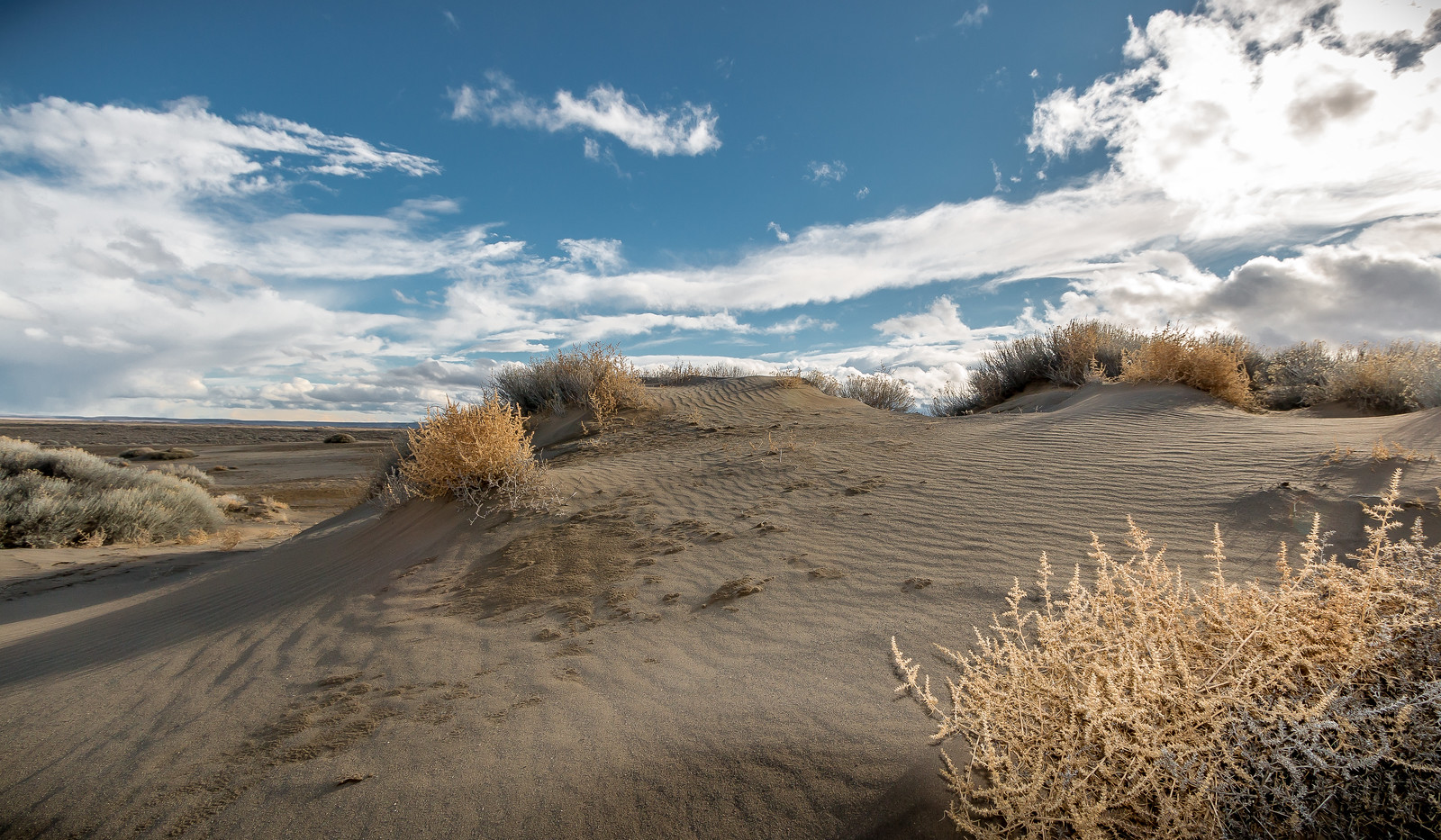The image depicts a vast, arid landscape reminiscent of a desert, characterized by extensive sand dunes and ripples shaped by the wind. The sand undulates in rolls and waves, evoking the movement of water, and it's surrounded by sparse, predominantly dead vegetation that appears brown, white, and grayish. Low hills and mounds dot the scenery, with one to the left forming a path between two elevations. Additional hills on the right are sprinkled with light shrubs and dry tumbleweed, possibly dark green in the distance. Small boulders are scattered across the sandy terrain. The horizon is a mix of gray and brown hues, blending into a medium blue sky filled with thick, rolling white clouds. The clouds also cluster near the lower part of the image, enhancing the desolate yet striking beauty of this desolate expanse.